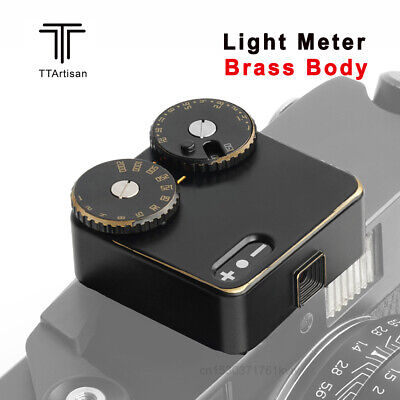This advertisement features a detailed product photo showcasing a light meter designed for Leica cameras. The device, made by TT Artisan, is mounted on a semi-transparent camera which gives a ghost-like effect. The light meter is a small, black square and boasts a brass body with exquisite gold detailing. On its top, it has two circular dials adorned with shallow teeth and gold numbers and trims. These dials are likely for adjusting ISO and shutter speed. The front of the device has a tiny lens or viewport accompanied by a plus and minus sign for exposure adjustments. The words "Light Meter" and "Brass Body" are written on the side, with "Brass Body" standing out in red text. The TT Artisan logo is prominently displayed, completing the sophisticated and functional design of this photographic accessory.